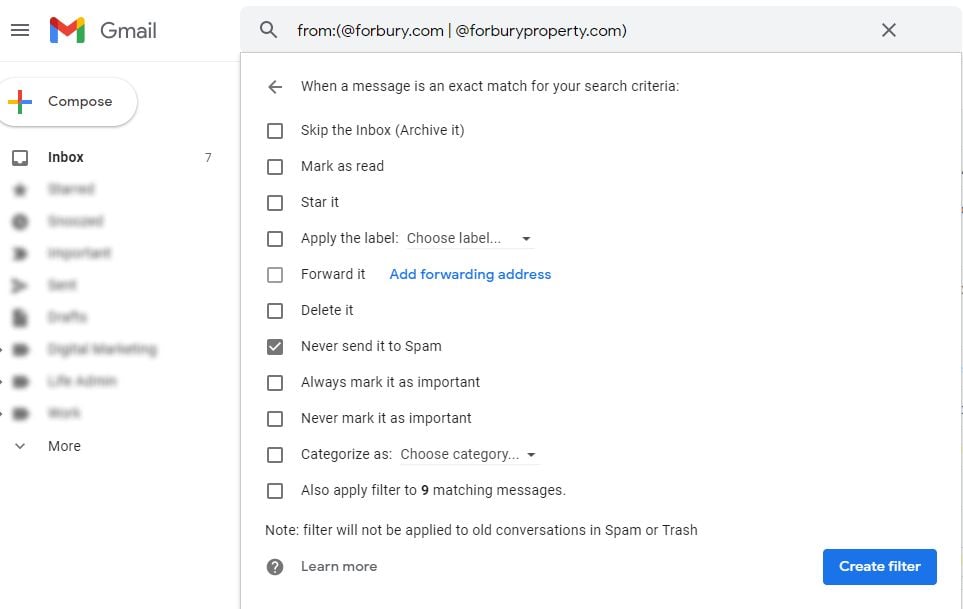This year in Gmail, the user interface includes a menu represented by three horizontal lines located in the top left corner. To its right is the Gmail logo, featuring an envelope adorned with red, blue, yellow, and green accents, followed by the word "Gmail." On the right side of the interface, there's a search icon accompanied by the text "from Poland (at forburry.com)" and a vertical line separating it from "at forburryproperty.com." On this same gray strip is an 'X' icon.

Below this strip, a notification bar appears with a left arrow icon. The message reads: "When a message is an exact match for your search criteria:" followed by a colon, which introduces a detailed list of filtering options. Each option is preceded by a checkbox, allowing users to select actions such as:

- Skip the Inbox
- Archive it
- Mark as read
- Star it
- Apply the label (with a dropdown to choose the label)
- Forward it
- Add forwarding addresses
- Delete it
- Never send it to Spam (this option is checked)
- Always mark it as important
- Never mark it as important
- Categorize it (with a dropdown to choose the category)
- Also apply filters to 9 matching messages

A note follows these options, warning: "The filter will not be applied to old conversations in Spam or Trash." Finally, a circle with a question mark icon provides a link to "Learn More."